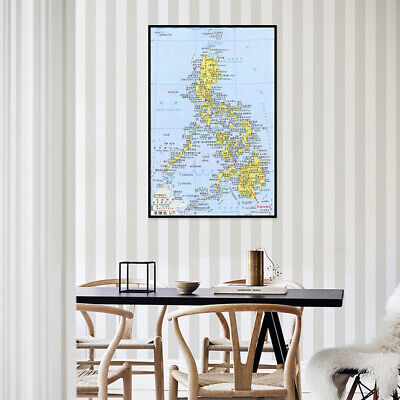The image is a digitally edited product photo of a framed map, placed in a dining room setting to give a sense of scale. The map features yellow landmasses, likely depicting various countries or cities, against a blue ocean, complete with labeled names and meridians. The map is encased in a black frame and positioned above a black dining table adorned with items including a white book, a small bowl, a candle, and a gold-colored cylindrical object. The table is surrounded by light brown wooden chairs, and to one side, a white fur-covered chair adds a touch of coziness. The background wall displays a distinctive striped pattern in yellow, white, and dark gray, enhancing the visual appeal of the setup.